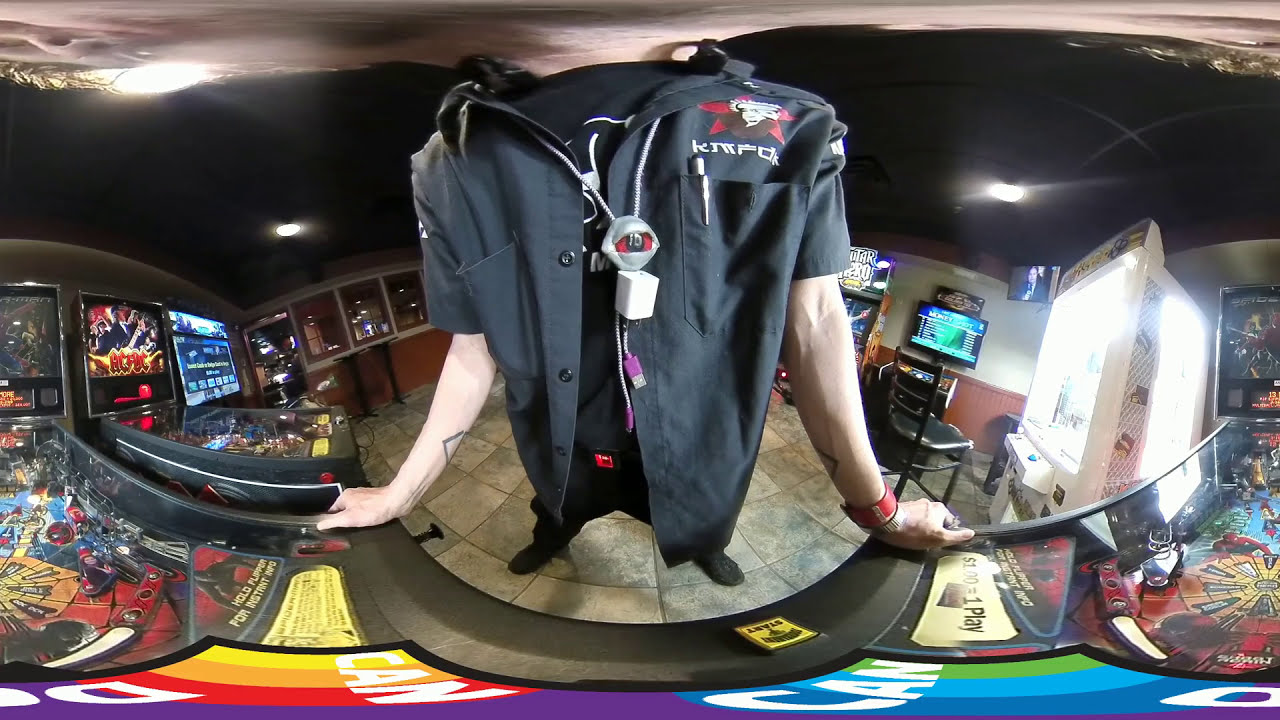This image captures a man leaning forward on a colorful pinball machine, his hands positioned on either side of the machine where the controls are typically found. Photographed from the neck down, his head is not visible. He is dressed in black, sporting a black t-shirt beneath an unbuttoned black shirt. Around his neck, he wears two chargers and a necklace adorned with a distinctive eyeball pendant. A pen is tucked into his left pocket, and his left wrist is adorned with a watch. Tattoos featuring half-triangle patterns decorate his forearms, suggesting a Caucasian appearance. The room, which resembles a gaming arcade or a sports bar, features a tile floor speckled with black, a wooden backdrop, and a high ceiling painted black. Various gaming machines, including pinball machines and a claw machine, populate the space. Additional features visible in the background include neon beer signs and a big screen TV in the top right corner of the image, enhancing the atmosphere of a lively entertainment setting.